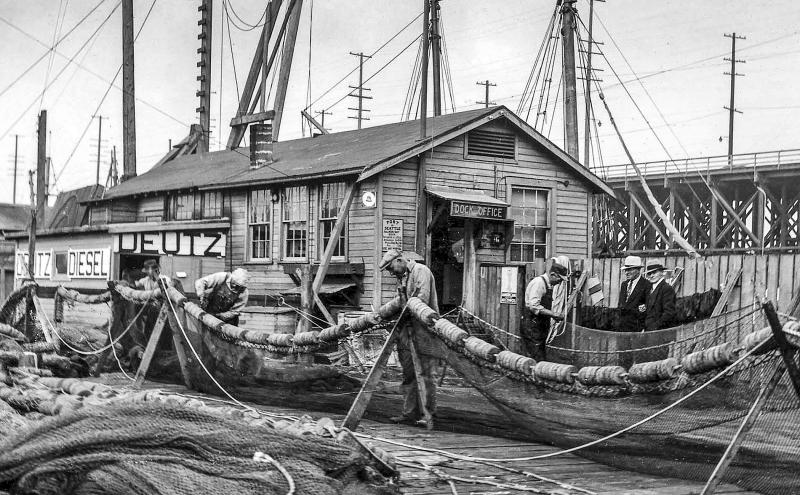The black-and-white photograph depicts a bustling dock area dominated by a wooden building labeled "Deutz Diesel" above its doors. The dock office sign is visible above a nearby entryway. The image features several men engaged in what appears to be labor-intensive work involving netting and ropes, possibly preparing or repairing fishing nets. Among the workers, dressed in work clothes, are a few men in suits who seem to be overseeing the activity. The background is filled with the vertical poles and rigging of ship masts, though no actual boats or sails are visible. The lower left corner of the image is cluttered with nets, adding to the maritime atmosphere.